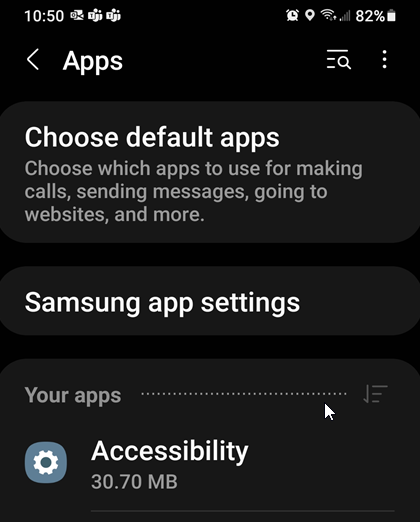The image is a smartphone screenshot featuring a predominantly black background with text in white and gray. At the top, there is a timestamp indicating "10:50". To the left of the timestamp is an email icon. Adjacent to this are icons representing two contacts, each marked with a number one. To the right of these icons are additional status icons including an alarm (indicating it is set), a location icon, a Wi-Fi icon, and a battery icon showing 82% charge.

Beneath this status bar, an interface with a left-facing arrow on the left, labeled "Apps", can be seen. To its right, there's a search icon followed by three vertical dots (typically indicating more options). The primary text on the screen reads:

"Choose default apps. Choose which apps to use for making calls, sending messages, going to websites and more."

Further down, the screen displays the heading "Samsung app settings" followed by the subheading "Your apps", underlined by a dotted line. Below this line is a settings wheel icon next to the word "Accessibility" along with a file size notation of "30.70 MB."

The overall content suggests a settings page where users can choose default applications and modify app settings specific to Samsung devices.